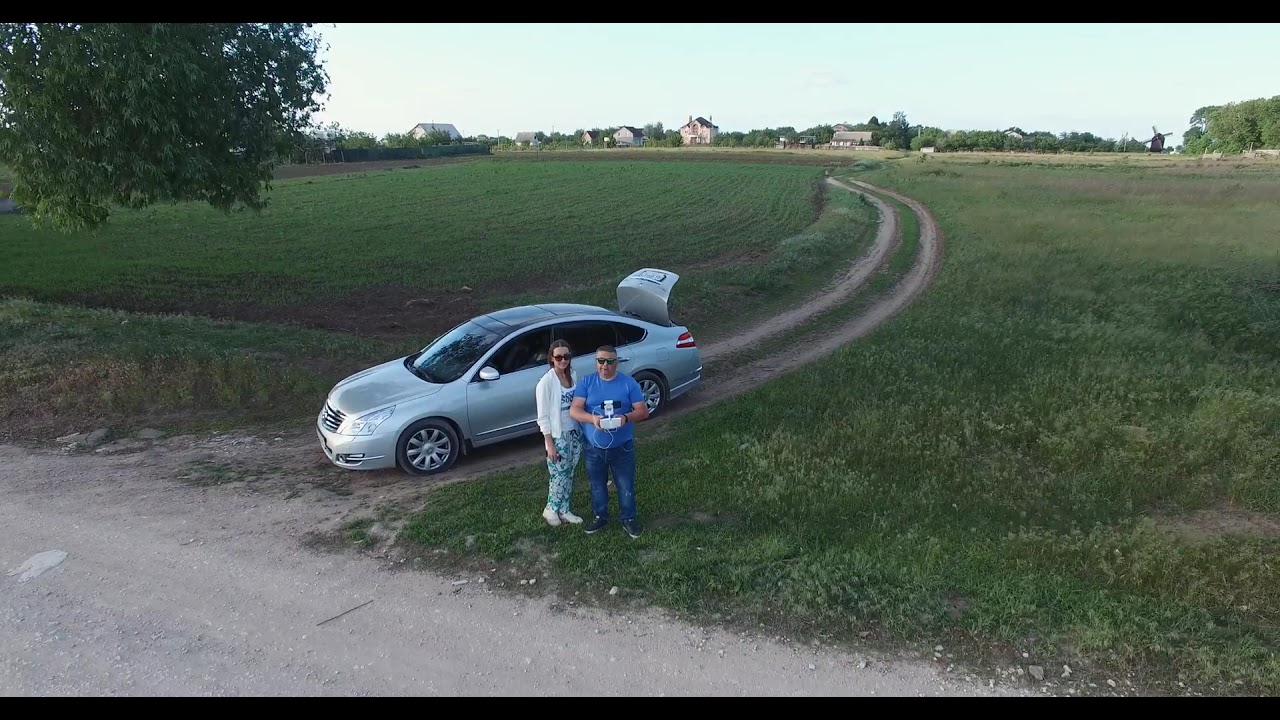In the image, a silver compact sedan with its trunk open is parked in a grassy field with visible tire tracks leading towards the camera. The setting seems rural, with a grayish dirt road occupying the lower left corner of the frame and extending into the green expanse of the field. Two individuals, a man and a woman, are standing in front of the car, looking directly at the camera as if posing for a picture. The man, positioned to the right of the screen, wears a blue T-shirt and jeans, and appears to be holding a white box resembling a drone controller. The woman, to his left, is dressed in a white T-shirt and floral print, white and blue pants. Both are wearing sunglasses. In the background, the horizon line reveals a series of small houses and trees under a light blue sky, suggesting daytime. The upper left corner features the leaves of a tree extending into the frame. The overall image is bordered by thin black lines at the top and bottom.